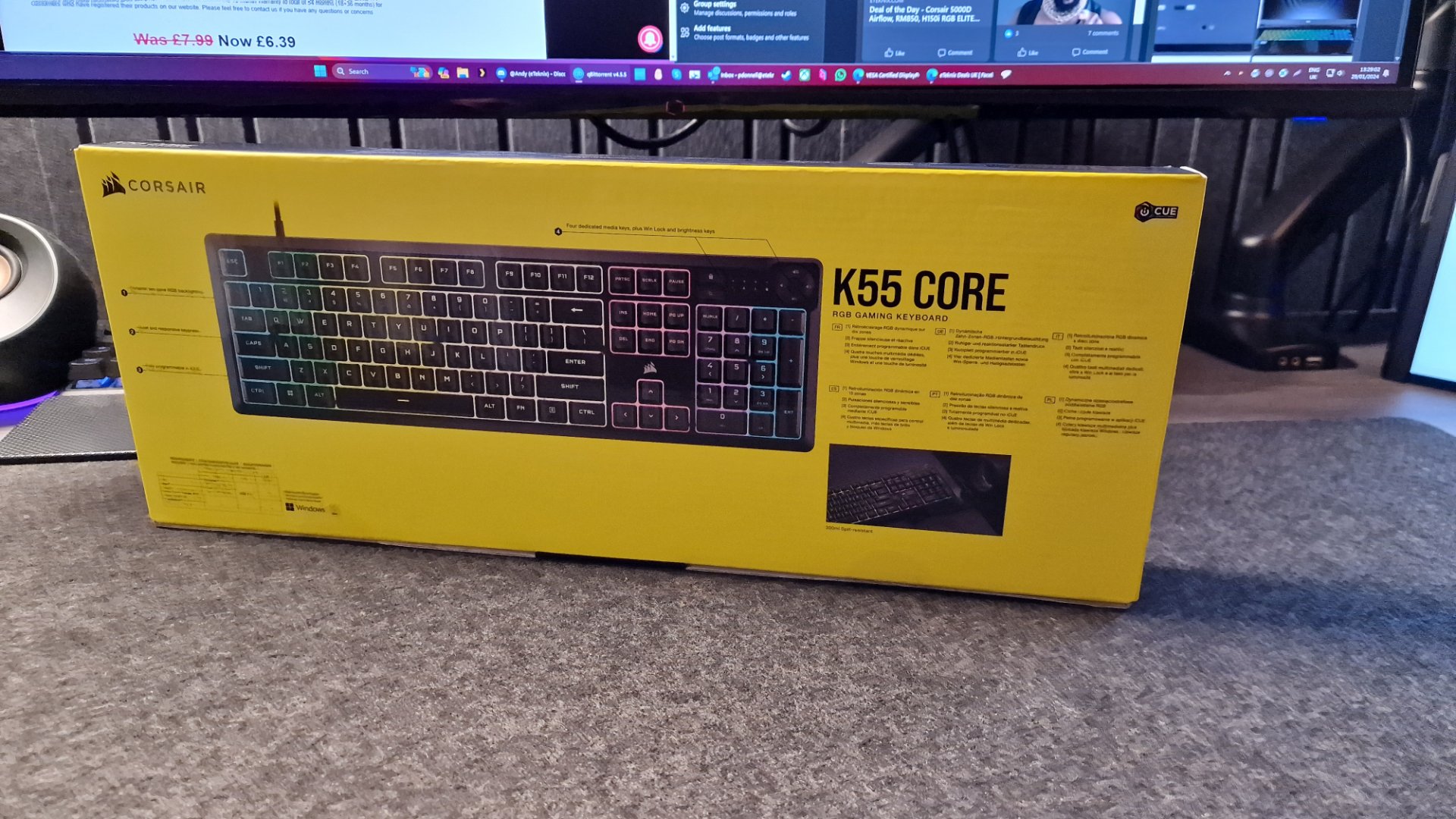This product photo captures a brand-new CORSAIR keyboard, still in its box, placed upright on a keyboard mat atop a brown wooden table. The box, which is prominently yellow at the top left corner showcasing the CORSAIR logo, is positioned at an angle towards the left. Dominating the front of the box is an eye-catching image of the keyboard illuminated in vivid colors: a gradient transitioning from blue on the left, to yellow, then pink, and back to blue. At the top right corner of the box, "K55 COR" is printed in large, bold letters. Just below this, six smaller boxes provide brief descriptions about the product. Towards the bottom right corner of the packaging, there is a small thumbnail image of the keyboard laid out on a flat surface. In the background of the image, above the keyboard, the bottom edge of a large, flat-screen monitor is visible.